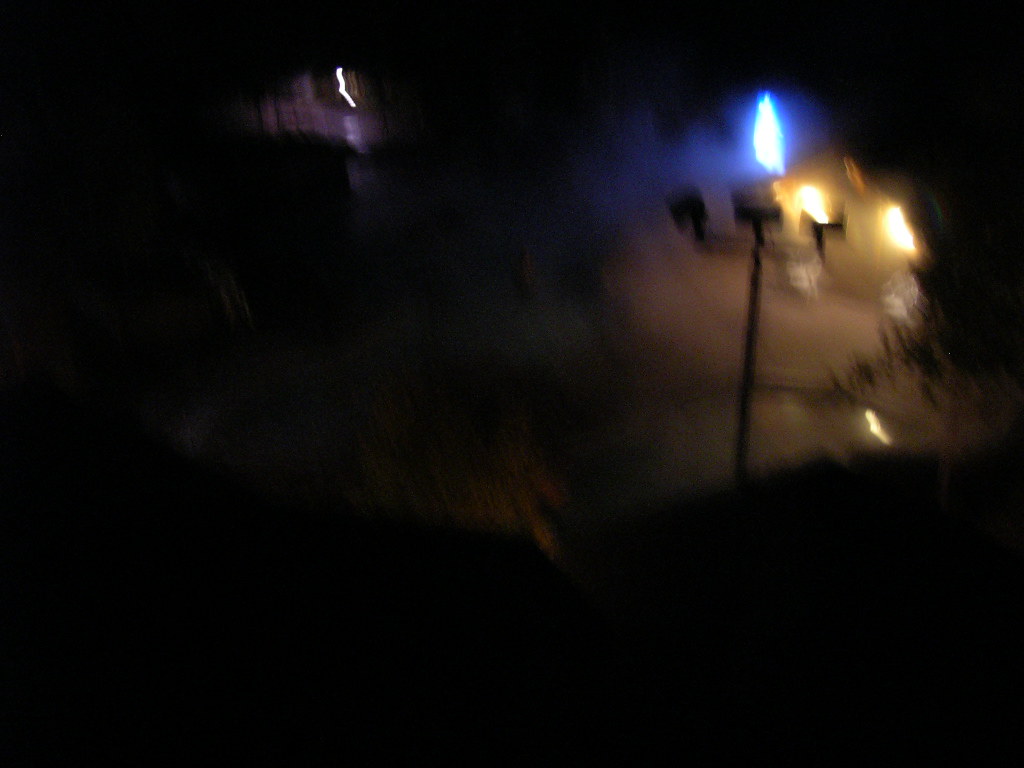This image features a dark and blurry scene dominated by a deep black background that covers approximately 40% of the lower section, left-hand side, and parts of the upper and right-hand edges. At the center, an opening reveals several elements. A silhouette of a green plant is visible toward the bottom, and a telephone pole, branching into three T-shaped structures, stands prominently in the middle. Distant light sources include two beams of yellowish-white light and one beam of light blue-white light, which emanates into a faint light blue background at the top right. The ground is a light brown, adding slight contrast to the darker tones. The right-hand side also features a few indistinct, blurry images of leaves, contributing to the scene's overall enigmatic and dim appearance.